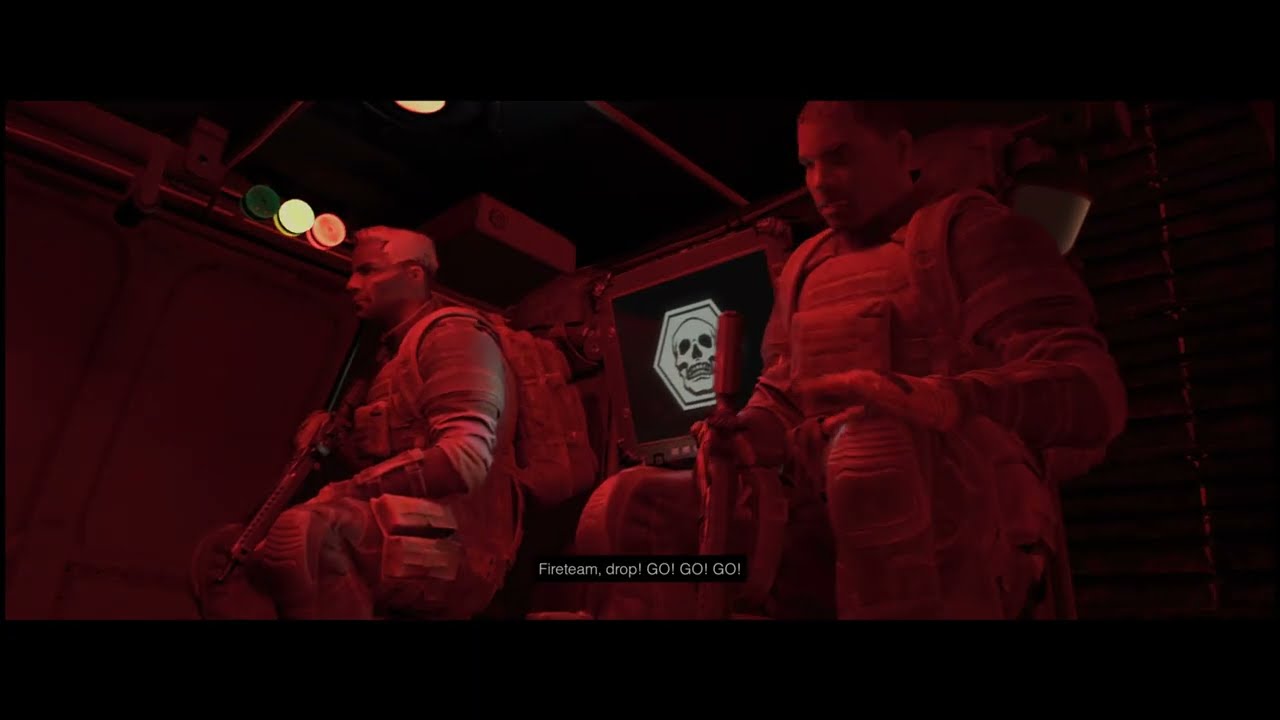The image is a detailed, digital screenshot from a video game, showcasing a tense scene steeped in red tones emanating from artificial lighting within a metallic transport vehicle. At its forefront, two adult male characters, seated and donned in military-style gear, including body armor, vests, knee pads, and backpacks, are the central focus. Both appear to be armed; the character on the left visibly holds a gun, while the character on the right's weapon is obscured. The figure on the left sports short, light-colored hair, contrasting with the seemingly bald character on the right. Dominating the dimly lit space behind them is a striking black screen displaying a white skull within a hexagonal border. Additional lighting is faintly visible in the upper left, comprising red, yellow, and non-illuminated green indicators. The bottom of the image is bordered by a black rectangle containing a bold, white caption that reads, "Fireteam, drop! Go, go, go!” This vivid and atmospheric representation captures the essence of a high-stakes moment within the game's universe.